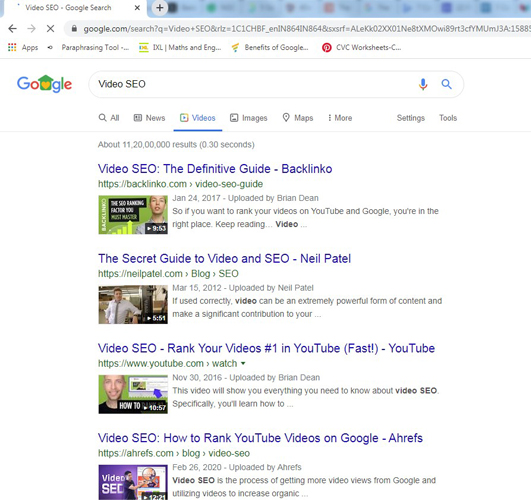This is a detailed caption for an image showing a Google search results page:

"In this screenshot of a Google search, the distinct Google logo is visible in the top left corner of the browser window. Below it, the search bar displays the query 'video SEO.' Beneath the search bar, there are several navigational tabs including 'All,' 'News,' 'Videos,' 'Images,' 'Maps,' and a menu with three vertical dots next to 'More,' as well as options for 'Settings' and 'Tools.' The 'Videos' tab is currently selected and highlighted in blue.

The search yielded approximately 11,200,000 results, displayed in just 0.30 seconds. Since the 'Videos' tab is active, all the listed results are video links, each accompanied by a small thumbnail preview. The top results include videos like 'Video SEO: The Definitive Guide' by Backlinko, 'The Secret Guide to Video and SEO' by Neil Patel, 'Video SEO: Rank Your Videos Number One on YouTube Fast,' and 'YouTube Video SEO: How to Rank Your YouTube Videos on Google' by Ahrefs.

This visually rich search result page consolidates video-focused SEO content from multiple expert sources, providing a quick visual reference for users interested in enhancing their video search engine optimization strategies."